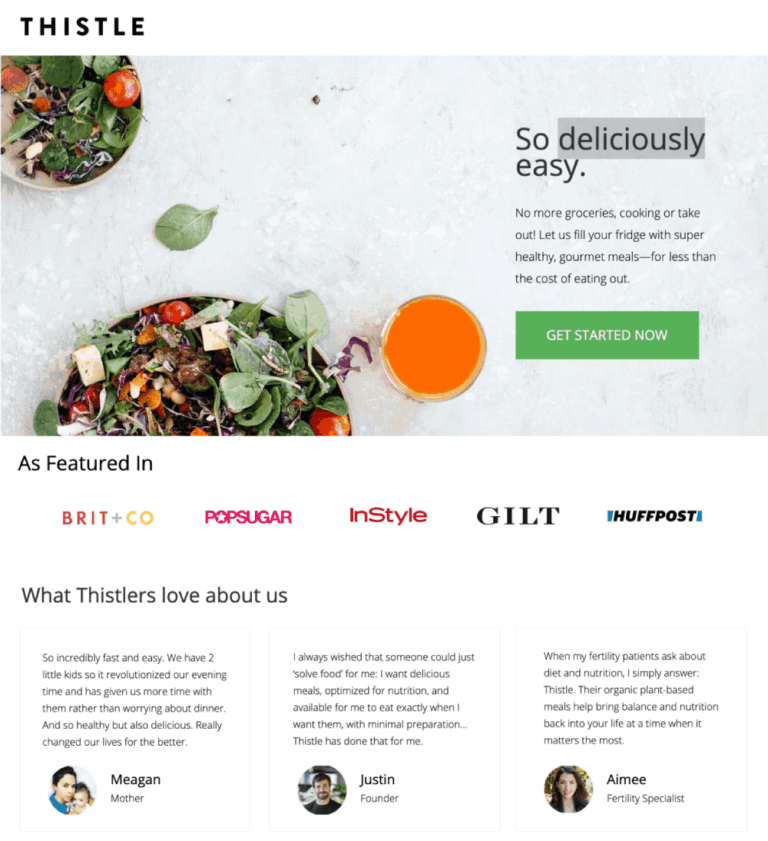This screenshot illustrates a website primarily designed as an advertisement for Thistle, a gourmet meal delivery service. The website's layout features a white background in the upper left corner, prominently displaying the brand name, "Thistle," in bold black font. Directly beneath this is an inviting photograph showcasing a white surface with two bowls brimming with fresh salad and a small cup of what appears to be French dressing.

To the right of the image, the website boasts a catchy slogan in gray font: "So deliciously easy. No more groceries, cooking, or takeout. Let us fill your fridge with super healthy gourmet meals for less than the cost of eating out." Below this promotional text, a green button with white font invites visitors to "Get Started Now."

Further down the page under the image, the website proudly presents an "As Featured In" section with logos of reputable media outlets such as Brit & Co, PopSugar, InStyle, Gilt, and the Huffington Post. This is followed by a section titled "What Thistlers Love About Us," which highlights customer testimonials. The first testimonial reads, "So incredibly fast and easy. We have two little kids, so it revolutionized our evening time and has given us more time with them rather than worrying about dinner. So healthy but also so delicious."

Overall, the website effectively combines attractive visuals and compelling text to promote Thistle's meal delivery service, positioning it as a convenient and nutritious alternative to traditional meal preparation.